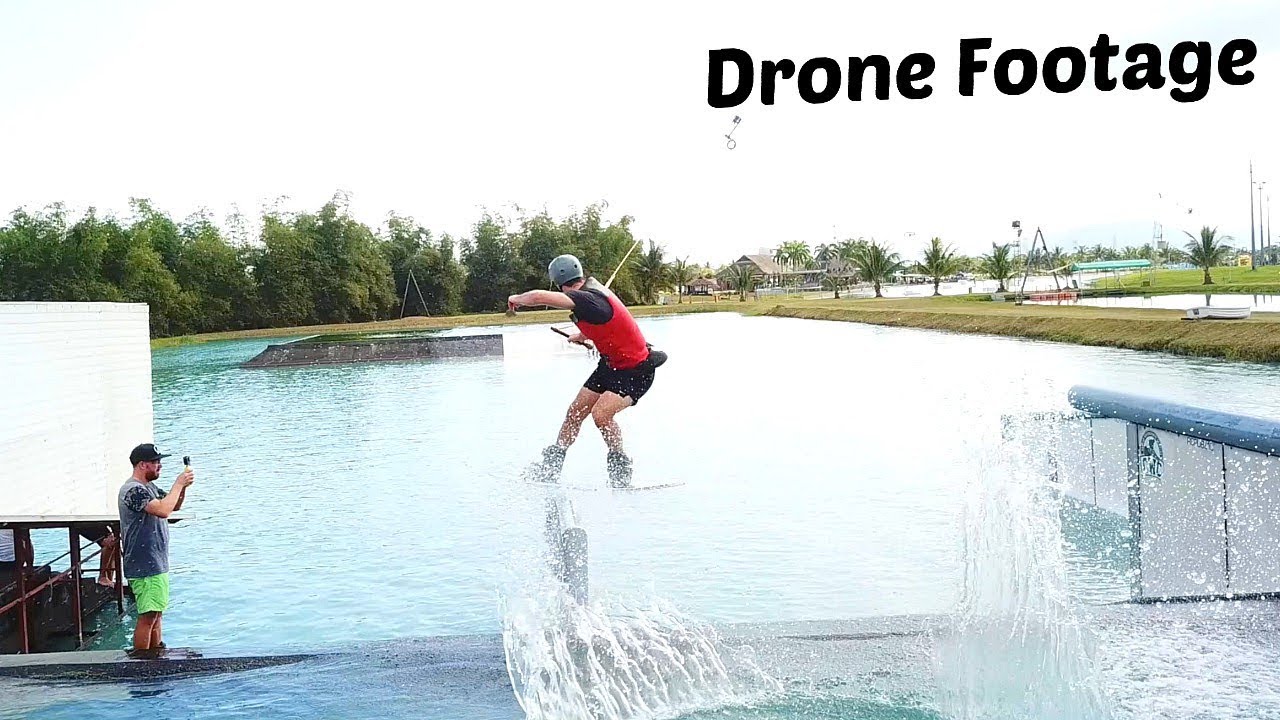In the color photograph entitled "drone footage," a man is seen water skiing on what appears to be a large lake or man-made pond. The setting is well-lit, suggesting it is daytime. In the middle of the image, the man is suspended in the air as he holds onto a water skiing line, creating a dynamic and intriguing focal point. On the left side of the photograph, another man is capturing the scene on his phone. This man is detailed with a black baseball cap, facial hair, a dark blue short-sleeved shirt, and green shorts. He is positioned in front of a white billboard. The background features lush greenery, including several palm trees and grassy areas, adding to the scenic, possibly tropical, ambiance. There is also a house visible, hinting that the location could be in Florida or a similar region. The photograph encapsulates a vibrant and lively lakeside activity with clear details of the surroundings.